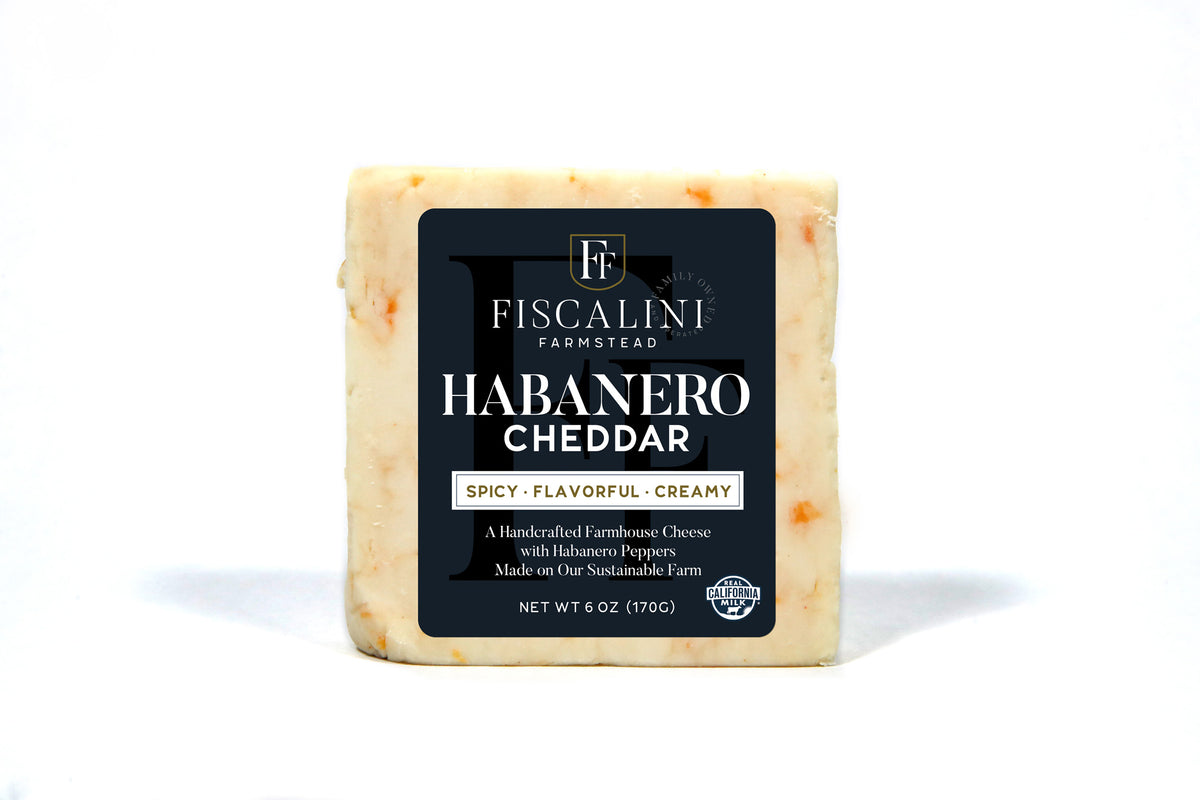This image features a block of cheese set against a white background, with a subtle light blue shadow beneath it. The cheese, a light yellow cheddar with visible orange and red flecks indicating the presence of habanero peppers, is tightly wrapped in plastic. Prominently displayed on the front of the cheese is a large black label in the shape of a shield with rounded corners.

The top portion of the label displays the brand name "FISCALINI FARMSTEAD" in bold, all caps white letters. Above the brand name is a small logo featuring an "FF." Centered on the label, also in bold, all caps white letters, are the words "HABANERO CHEDDAR." Underneath this, in brown text against a white rectangular background, it reads "Spicy. Flavorful. Creamy."

Further details are provided below in smaller white text: "A handcrafted farmhouse cheese with habanero peppers made on our sustainable farm." The weight of the cheese is specified as "Net Weight 6 oz (170 G)." Additionally, in the lower right corner of the label, there is a small circular California Milk logo with an image of a cow, affirming its quality and origin.

The cheese's visually inviting appearance, with its subtle shadows and vibrant pepper flecks, promises a spicy yet creamy flavor experience.